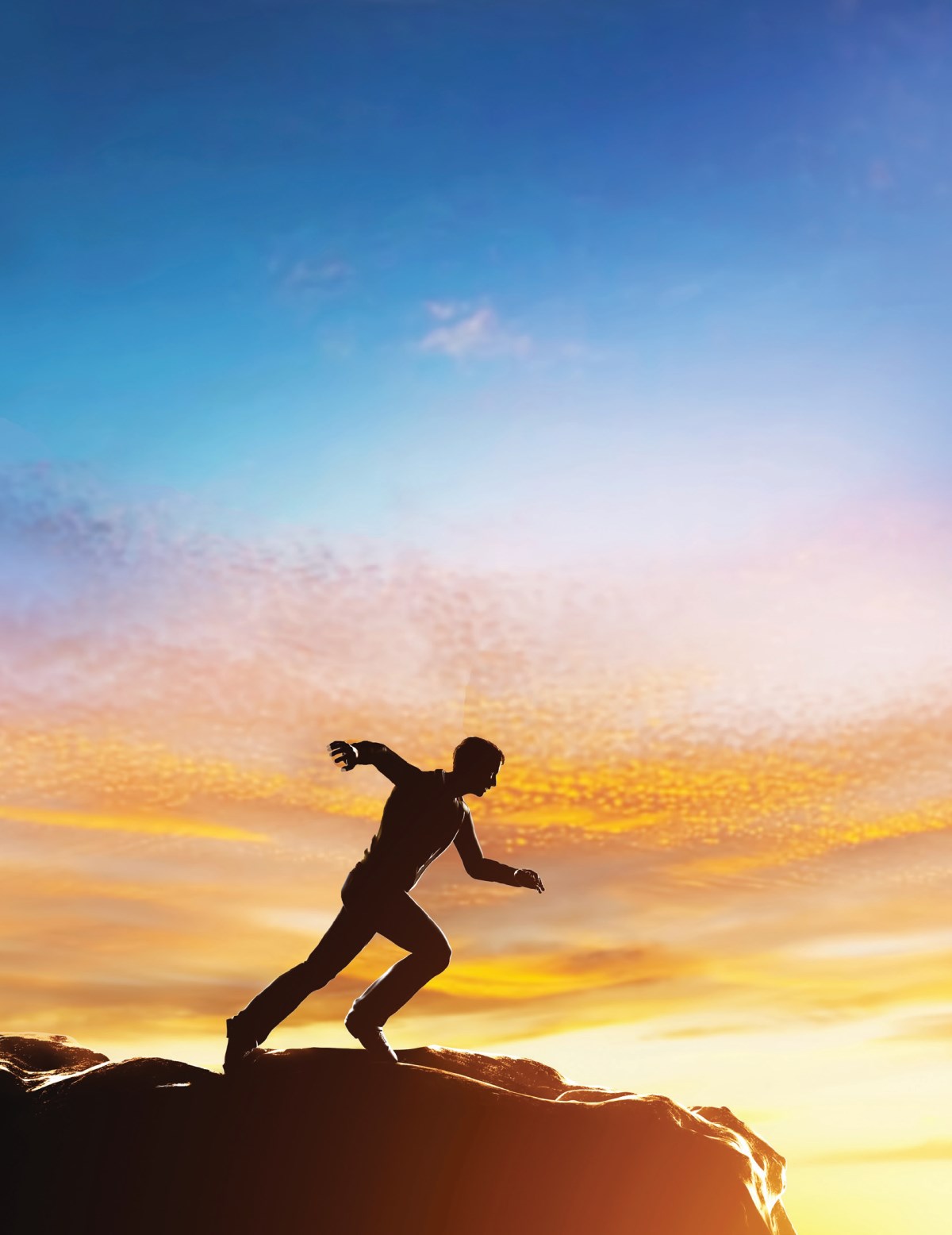The image depicts a silhouette of a young man running on what appears to be a somewhat curvy and possibly jagged rock or cliff. The runner, captured in mid-stride with one leg bent in front of the other and arms extended out to the sides, appears to be moving towards the right side of the image. The sky above him is a stunning gradient of colors: it starts with bright blue at the top and transitions into a bright yellow and hints of pink near the horizon, suggesting the sun has just set. There are also a few wispy clouds visible in the sky. The overall effect casts the figure in shadow, making it difficult to discern specific details, but creating a dramatic and striking silhouette against the vibrant evening sky.